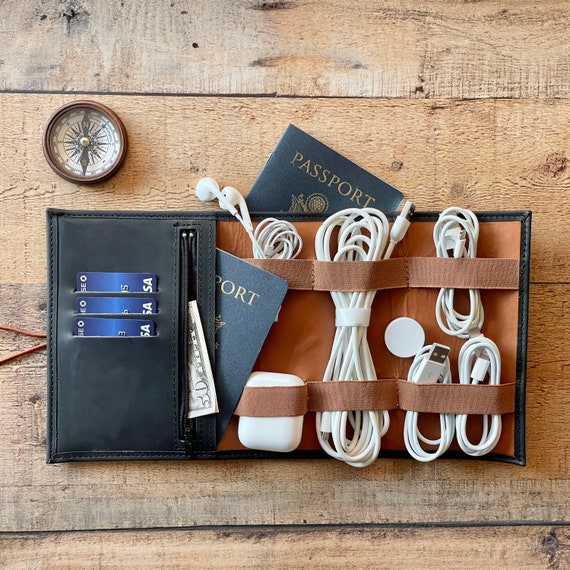This image shows a detailed flat lay of travel essentials neatly organized in a black wallet with brown lining and elastic straps. The wallet holds two passports, three credit cards, and a $50 bill folded and tucked into a zipper pocket. There's a pair of Apple earbud headphones and several neatly wound Apple charging cords secured under elastic straps. Additionally, a pair of white AirPods are included in the setup. To the top left of the wallet is a vintage-looking compass, small enough to fit in the palm of a hand. All items are arranged on a warm-toned, raw, unfinished wooden plank, giving the scene a rustic and organized feel.